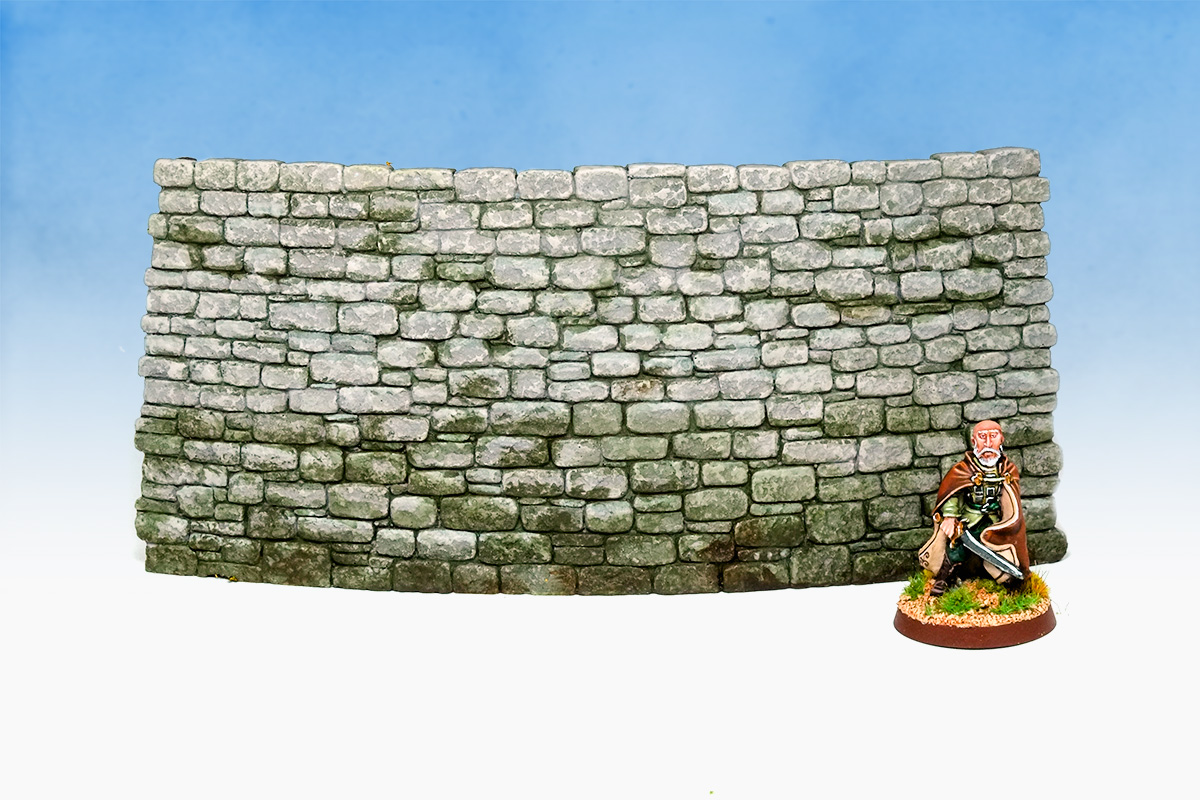The image appears to be a detailed prop for a tabletop role-playing game. Central to the scene is a meticulously crafted stone wall, showcasing extensive weathering and moss particularly concentrated at the bottom, transitioning to a lighter color towards the top. The wall occupies about three-quarters of the image horizontally and sits against a gradient background that shifts from white at the bottom to blue at the top.

In front of this wall, positioned strategically on the bottom right corner, stands a highly detailed figurine of an older man. This miniature figure has a bald head and a white beard, donned in a reddish-brown cloak and what appears to be leather armor. He is also holding a silver sword. The figure stands on a brown base that simulates gravel, accentuated with tufts of grass and weeds, enhancing the realism. The detailed craftsmanship of both the wall and the figure underscores the intricate artistry characteristic of high-quality tabletop gaming props.